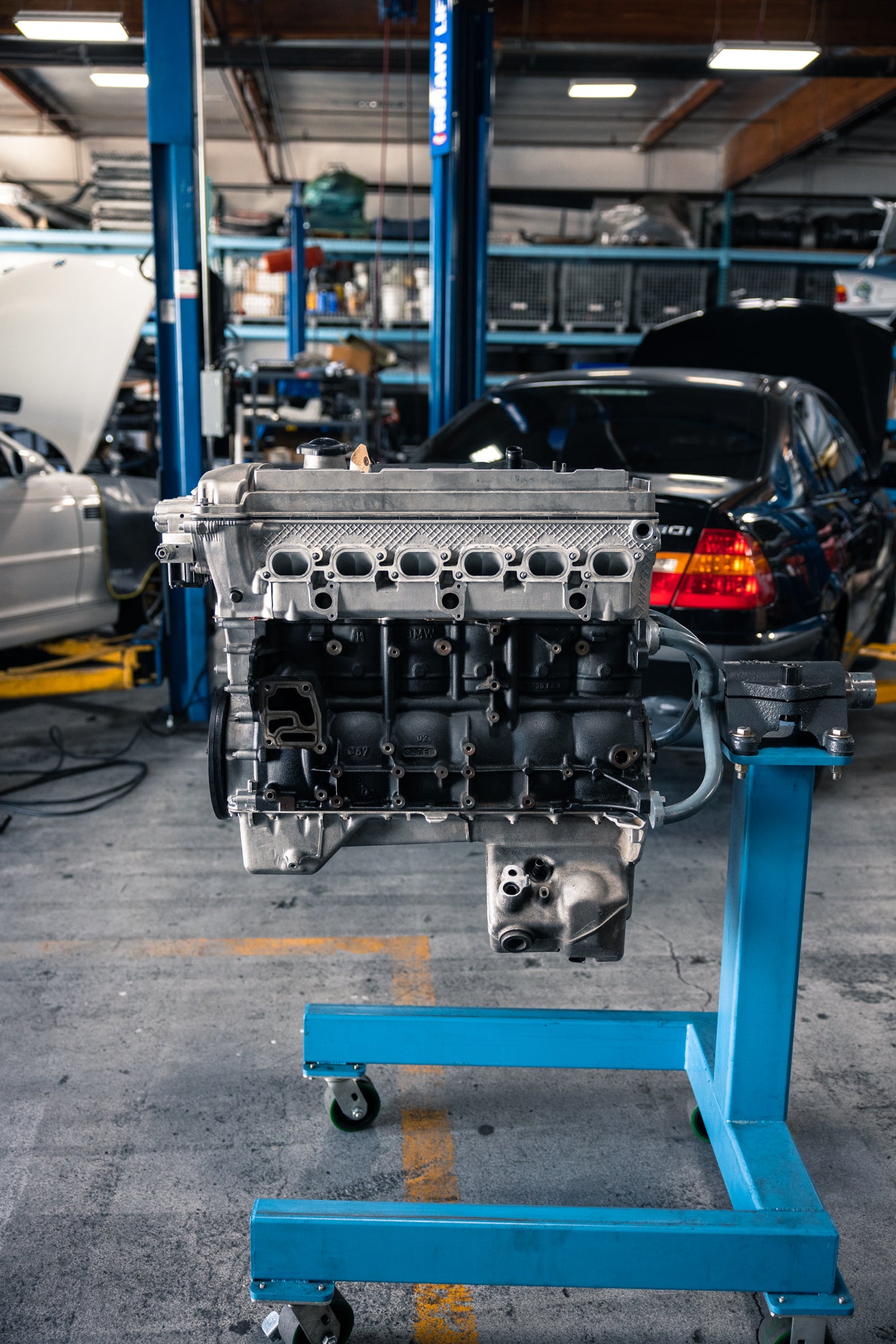The image captures the interior of a bustling car repair garage. In the foreground, prominently positioned close to the camera, sits a large engine mounted on a blue rolling engine lift, offering a detailed view of its silver top and black bottom. This apparatus, supported by four wheels, suggests it's likely used to diagnose and inspect the engine for any issues, such as cracks or other problems.

Moving to the midsection of the image, there are two blue pillars that run vertically, segregating different bays. To the left, under a yellow lift, is a white or possibly gray car with its hood up, indicating ongoing engine work. Adjacent to this, to the right of the blue pillars, is a black BMW, also on a lift with its hood open, seemingly being worked on as well.

The background, though slightly blurry, reveals more details of the garage's interior. Shelves stocked with tools and various car parts line the back wall. Overhead, fluorescent lighting brightly illuminates the space. The floor, made of concrete, features markings delineating different working bay areas. The setting is meticulously organized, with the blue shelving, pillars, and pneumatic equipment adding a cohesive aesthetic to the workspace. Very subtly in the background, a car that somewhat looks like the rear end of a Volvo is parked, providing depth to the scene.